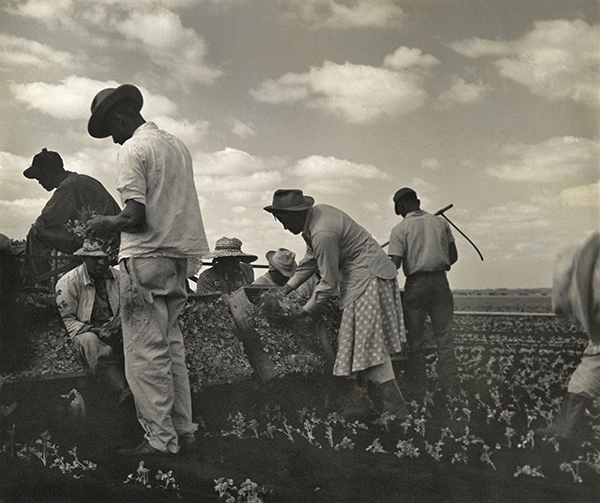This is a square, old black and white photograph capturing about ten individuals working diligently to harvest crops on a farm. Under a partly cloudy sky, these farmers, dressed in a variety of practical work attire, can be seen engaging in the laborious process. Most are either standing or seated around a machine in a dirt-laden area, indicating the use of some mechanized aid in their task. 

In the foreground, a man in a white shirt and worn trousers wears a hat to shield himself from the likely warm sun. Nearby, a woman stands out in a polka-dotted skirt and a brimmed hat, contributing to the harvest as she loads crops into wooden crates. Several other workers, both men and women, are similarly attired with broad-brimmed straw hats and are either standing or seated, tending to the crates and assisting in moving them once filled.

The machinery mentioned resembles a tractor or similar vehicle, with individuals both feeding crops into it and sitting atop it or behind it, possibly aiding in the transportation of full bins. The crops, planted in orderly rows, stretch into the backdrop of the image, highlighting the expansive farmland. Though faces and details are not clearly visible due to the photograph's age and orientation of the individuals, their dedicated efforts under the sun are evident in this timeless depiction of agricultural life.